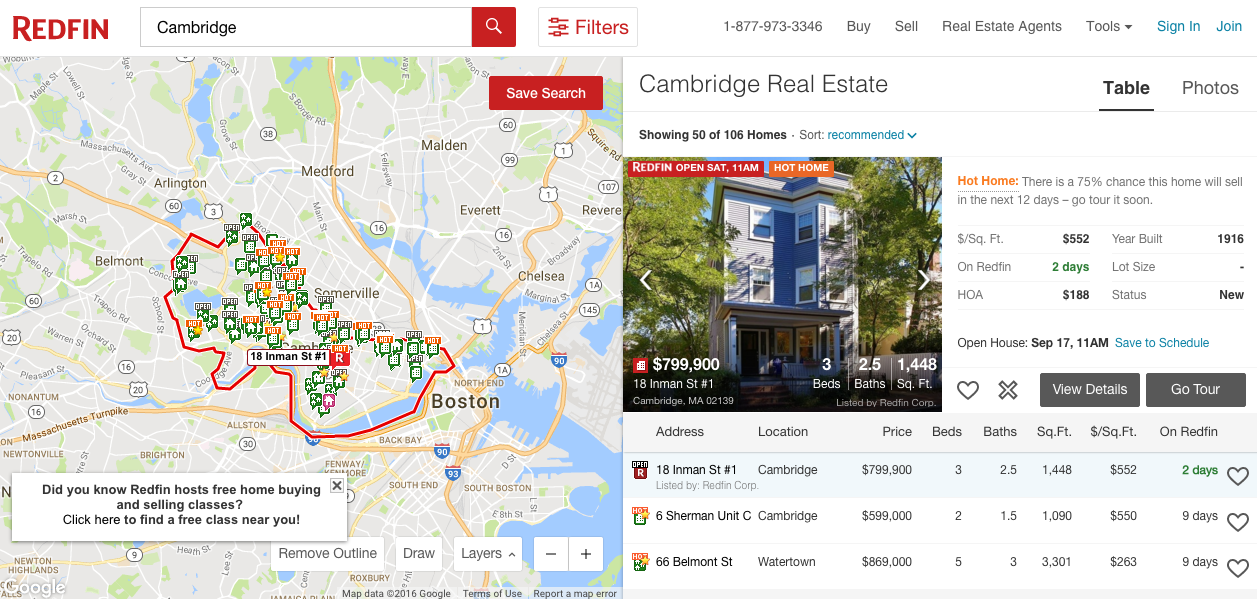This screenshot captures the user interface of Redfin, a prominent real estate website, focusing on a search within the Cambridge area of Massachusetts. 

At the top left of the image, the Redfin logo, prominently red, marks the header. Adjacent to this are a search box and filter section seamlessly integrated on the same row. This header also includes a phone number, real estate agent tools, and options to sign in or join the platform.

Below the search box on the left side, a detailed map of Boston is displayed. Overlaid on this map is a white pop-up that reads, "Did you know Redfin hosts free home buying and selling classes? Click here to find free classes near you." 

On the right side of the screenshot, a comprehensive list of Cambridge real estate options is presented. Dominating this list is an image of a townhouse labeled as a hot home, priced at $799,900. This property is advertised as being open for viewing on Saturday at 11 AM. Additional details include its address, three bedrooms, two bathrooms, and a total area of 1,448 square feet.

Below this main listing, additional addresses of available real estate in the Cambridge district are provided. Each listing includes relevant information such as location, price, number of bedrooms and bathrooms, square footage, and the number of days the listing has been on Redfin. 

These details are set against a dark gray background and are accompanied by interactive elements such as "View Details" and "Go Tour" buttons, as well as heart and X icons for favoriting or dismissing listings.